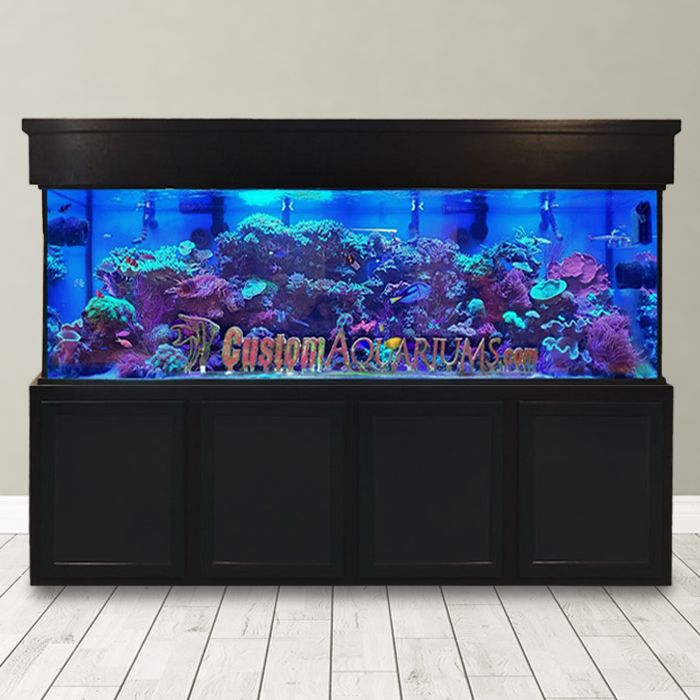You are looking at a color photograph of a very large, custom aquarium positioned against a light gray or beige wall and situated on a white wood floor with visible grain, giving it a white-wash, gray-white appearance. The aquarium sits on a substantial black base featuring four panels or doors. The aquarium itself is filled with clear blue water and is vividly illuminated, showcasing a variety of tropical fish, including yellow, blue, and orange species as well as some exotic-looking creatures and corals. One notable feature inside the tank is a large rock formation that could be coral or volcanic rock. At the top of the tank, there is a dark wooden hood. Across the front of the tank's glass is the branding "customaquariums.com."